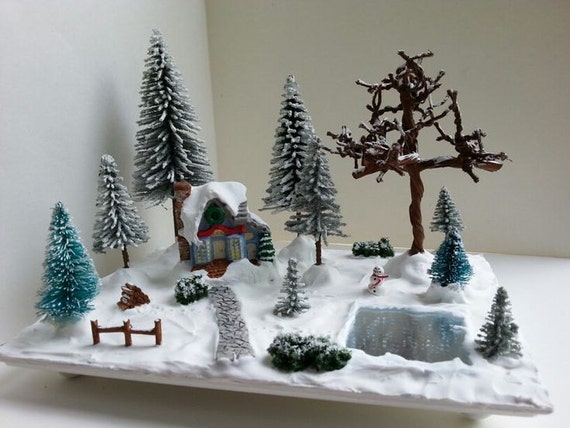The photograph captures a detailed miniature Christmas village set on a white table against white walls, enveloped in a snowy landscape. The scene features several frosted pine trees of varying heights, alongside a few barren trees, one prominently placed in the background with sparse branches and casting shadows on the wall. The centerpiece is a quaint miniature house on the left, characterized by its yellow door and a green wreath above it, its roof blanketed in snow. In the forefront of the display, there is a snowman adorned with a red scarf and buttons, positioned near an iced-over lake that hints at a possible ice-skating area. A pathway meanders through the scene, leading to the house and flanked by a small, three-post fence. Notably, a pile of about 15 firewood logs rests nearby. Additional elements include a green tree lying on the ground, a bush, and various winter decor items, all contributing to the festive atmosphere. The overall color palette incorporates white, brown, green, red, yellow, blue, black, and silver, creating a vivid and intricate winter wonderland.